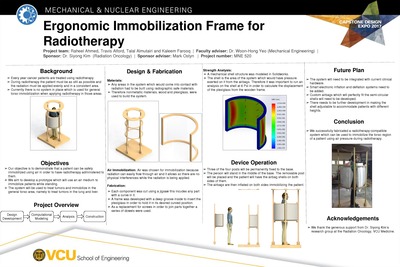This detailed informational sheet from the VCU School of Engineering, specifically the Department of Mechanical and Nuclear Engineering, is designed in a landscape format. It features a prominent black horizontal bar across the top with white text that reads "Mechanical and Nuclear Engineering". Within this bar, on the left side, is the VCU logo characterized by a blue background and a white sun motif. On the top right corner, there's an abstract, multi-colored logo, possibly related to a capstone expo, featuring shades of olive, gold, rust, silver, and blue.

Below this header, the central theme "Ergonomic Immobilization Frame for Radiotherapy" is clearly highlighted in bold black text. Accompanying this heading is a wealth of detailed text explaining the project, including a brief background, design and fabrication processes, the future plan, objectives, project overview, device operation, and acknowledgments. The sheet is visually enriched with several images, some in full-color and others in illustration, depicting various elements of the project. These images are arranged in a structured format, with three color illustrations side by side, followed by an additional illustration and a color photograph beneath, each accompanied by heading text in bold with descriptive smaller text.

At the bottom left corner of the sheet, the VCU branding is stamped in gold color with the words "School of Engineering" in small black text beside it, encapsulating the professional and educational context of the content.